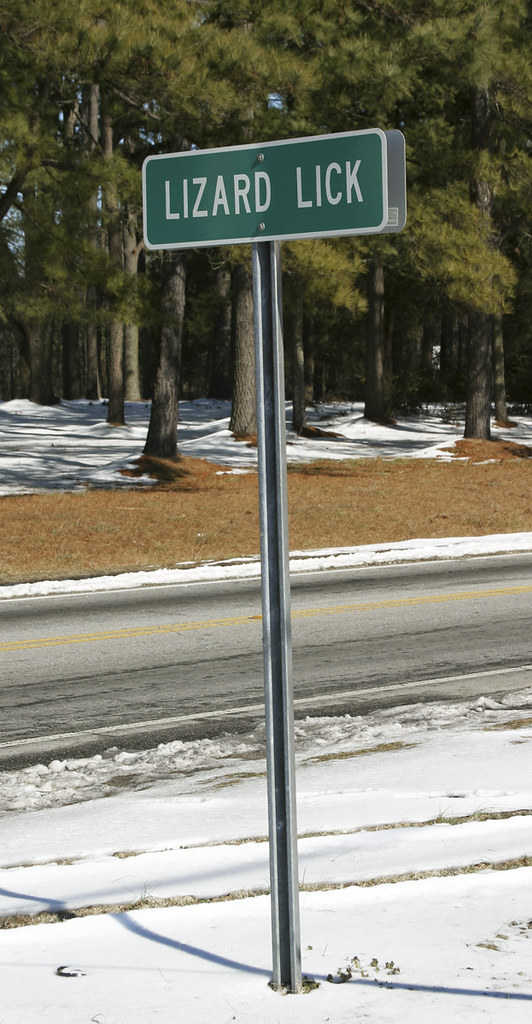A realistic winter scene unfolds in this photograph taken outdoors. A gray asphalt road, marked by a yellow center line, stretches through the image, flanked by snow-covered ground on either side. The snow reveals worn paths where the underlying grass is visible. On the right side of the road, a metal pole is embedded in the snow, supporting a green sign with a white border. The sign reads "Lizard Lick" in bold white letters. Across the street, brown mulch mingles with patches of snow, giving way to a grove of light brown tree trunks. These trunks are adorned with a plethora of leaves, and through their branches, a clear blue sky is visible, adding a touch of color to the wintry landscape.